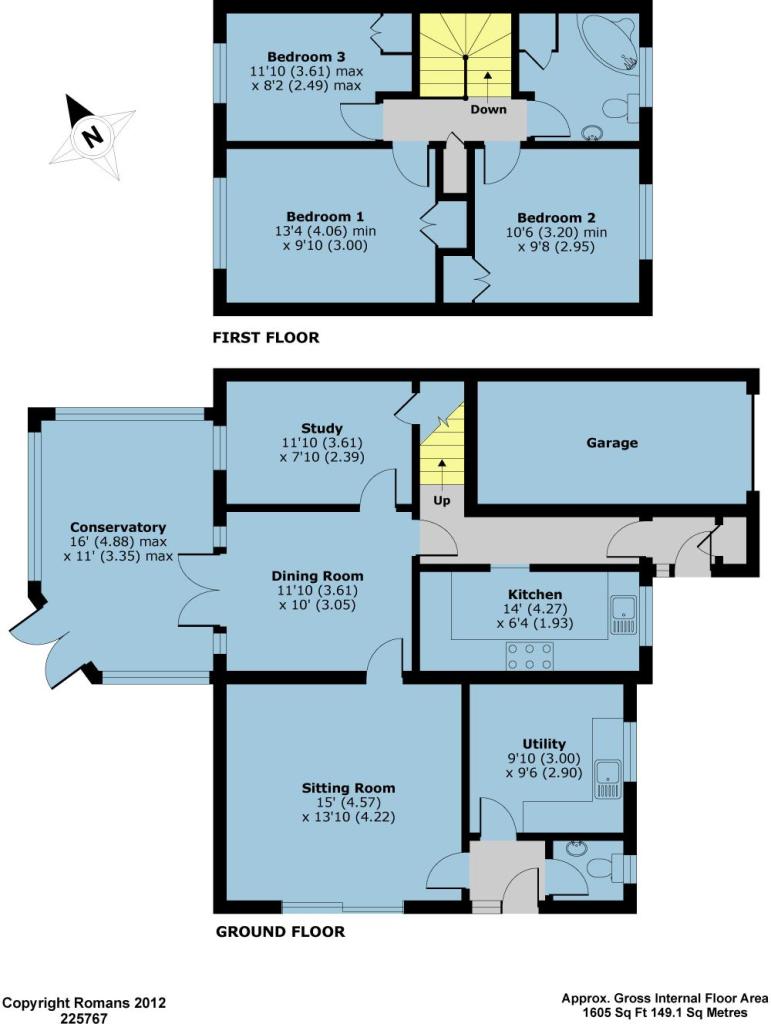The floor plan for a house, with a gross internal floor area of approximately 1600 square feet (149.1 square meters), is depicted in detailed schematic form. The house layout, attributed to Romans 2012 copyright 225767, features rooms illustrated in light blue and exterior walls demarcated by thicker black lines. Interior walls are marked with slightly thinner black lines, while the stairs are highlighted in a tannish color for distinction.

Starting on the ground floor, an entry door is positioned at the front on the right-hand side. Upon entering, there is a small bathroom immediately to the right and a utility room straight ahead. Moving left from the entryway leads into the sitting room. Adjacent to the sitting room is the dining room, which provides access to a conservatory on the left. Exiting the conservatory returns you to the dining room, from where you can enter the study. Turning right in the study leads to the hallway, which features a staircase leading to the upper floor. It is unclear how the garage is accessed, as no door is marked for it on the plan.

On the second floor, there are three bedrooms: two located at the front and the third situated at the back of the house. Additionally, there is one bathroom equipped with a tub, and the staircase connecting the floors is also present on this level.